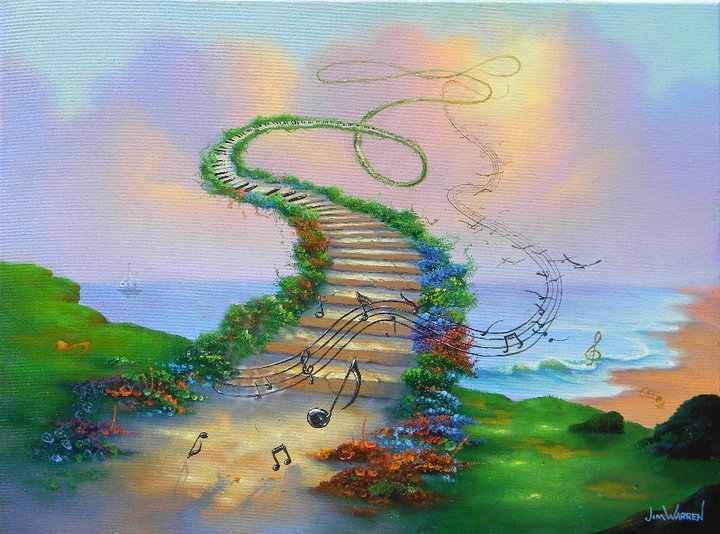The painting primarily features lush green hues with touches of blue and red accents. In the bottom right-hand corner, the artist's signature, "GM Warren," is visible. The foreground showcases a verdant cliffside abundant with grass, leading to a unique and imaginative "stairway to heaven." This stairway, composed of a natural pathway rather than cement or marble, ascends towards the sky, bordered by vibrant red and blue flowers. As the pathway rises, it seamlessly transforms into a piano keyboard, with a musical score meandering alongside it from the start of the stairs, creating a harmonious blend of nature and melody.

Beyond the cliffside, the painting reveals a serene shoreline with gentle waves lapping at the sand. The ocean is painted in rich blue tones, while the sky above is dotted with soft clouds. On the left side of the painting, a small boat rests on the horizon, adding a touch of tranquility to the overall composition. The scene masterfully combines elements of fantastical whimsy with the serene beauty of nature.